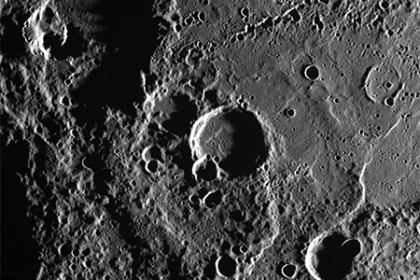This close-up photograph of the moon's surface, likely taken from outer space, captures the stark, cratered landscape in striking detail. Dominated by varying shades of gray, the image reveals a textured terrain marked by numerous craters of different sizes and shapes – from massive, near-perfect circles to smaller, jagged-edged indentations. In the top left corner, a significant black canyon or valley punctuates the landscape, while another canyon appears on the top right. The photo shows areas of raised terrain, including one notably circular elevated region. The surface has a rough, clay-like appearance with sunlit reflections creating subtle white highlights against a predominantly dark gray and black backdrop.